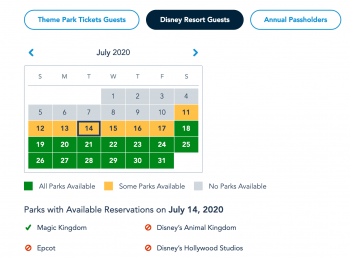The image depicts a reservation calendar for Disney parks in July 2020, tailored for different types of guests. The interface is divided into sections:

1. **Header Options**:
   - **Left Option (Blue)**: "Theme Park Tickets Guests".
   - **Middle Option (Black with White Text)**: "Disney Resort Guests".
   - **Right Option (Blue)**: "Annual Passholders".
   
2. **Calendar Display**:
   - The calendar is set to July 2020.
   - **Color-coded Dates**:
     - **Gray**: No Parks Available (1st to 10th).
     - **Yellow**: Some Parks Available (11th to 17th).
     - **Green**: All Parks Available (18th to 31st).
   - The 14th of July is highlighted with a dark blue square, indicating it is selected.

3. **Legend** (below the calendar):
   - **All Parks Available**: Green.
   - **Some Parks Available**: Yellow.
   - **No Parks Available**: Gray.

4. **Parks with Available Reservations on July 14, 2020**:
   - **Magic Kingdom**: Available (indicated by a green checkmark).
   - **Epcot**: Not available (indicated by a red cancel icon).
   - **Disney's Animal Kingdom**: Not available (red cancel icon).
   - **Disney’s Hollywood Studios**: Not available (red cancel icon).

The entire layout is set against a clean white background, providing a clear and organized view for the user.